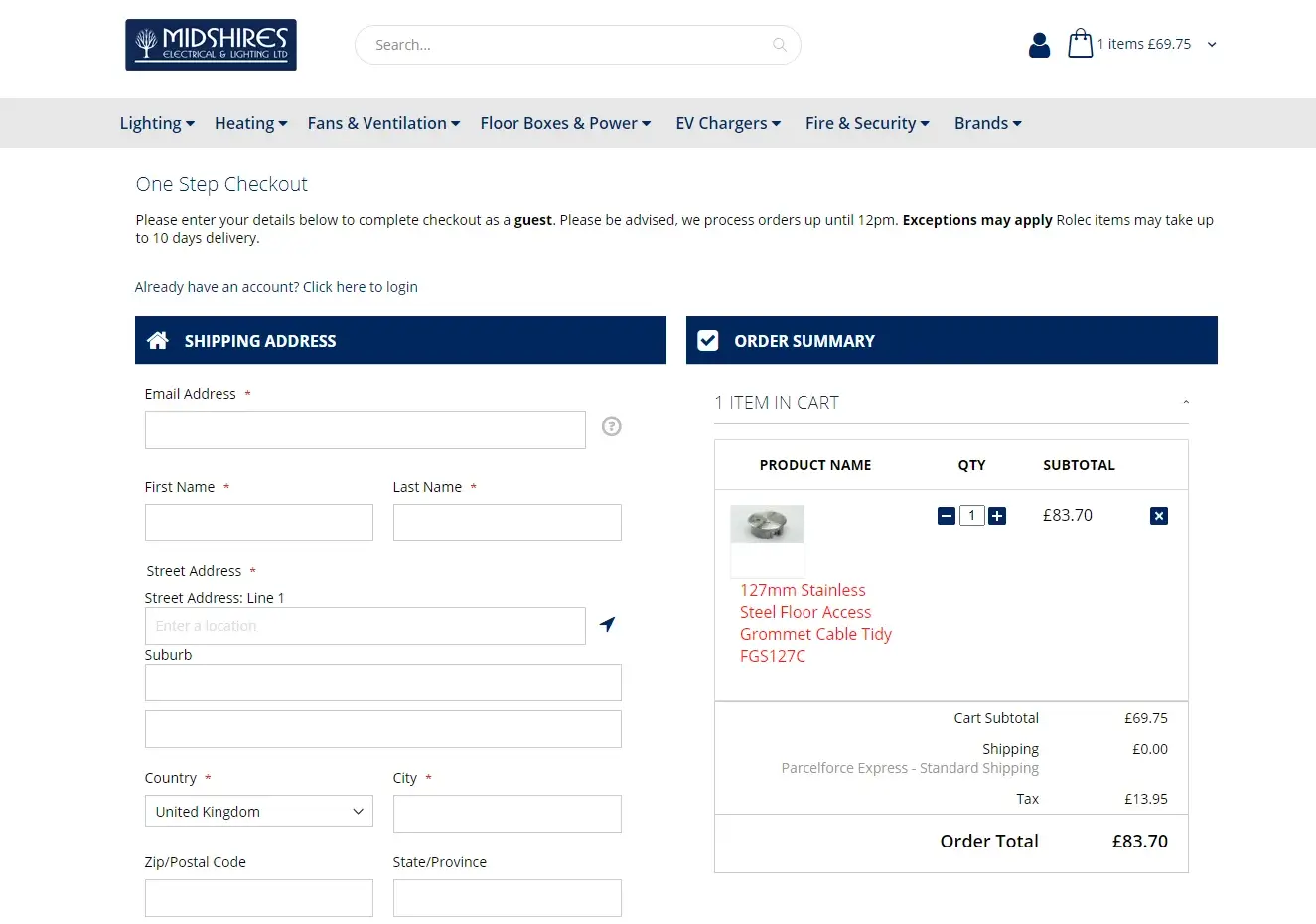The image is a screenshot of the Midshires Electrical and Lighting LTD website, characterized by its minimalist design with a white background. In the top left-hand corner, a small rectangle with a dark blue background features the company’s name in white text: "Midshires Electrical and Lighting LTD." Below this, a thin horizontal line separates the logo from a simple icon of a barren tree to the left.

At the top of the webpage, there is a search bar. Next to it, the shopping cart icon indicates one item with a total amount of £69.75. A gray navigation bar runs across the top, providing menu options for various categories including Lighting, Heating, Fans and Ventilation, Floor Boxes and Power, EV Chargers, Fire and Security, and Brands.

Underneath the navigation bar, a section titled "One-Step Checkout" instructs users to enter their details to complete the purchase as a guest. This section emphasizes the word "guest" in bold. Additional bold text advises customers that orders are processed until 12 p.m., with possible exceptions, and that Rolec items may take up to 10 days for delivery. A prompt for existing account holders to log in is also included.

The checkout section is divided into two columns. On the left, users are asked to input their shipping address details, including email address, first name, last name, street address, suburb, country, city, postal code, state, and province. On the right, the order summary lists the product details, including the item name (127mm Stainless Steel Floor Access Grommet, Cable Tidy), quantity, and subtotal. The total cost, including shipping and tax, is £83.70.